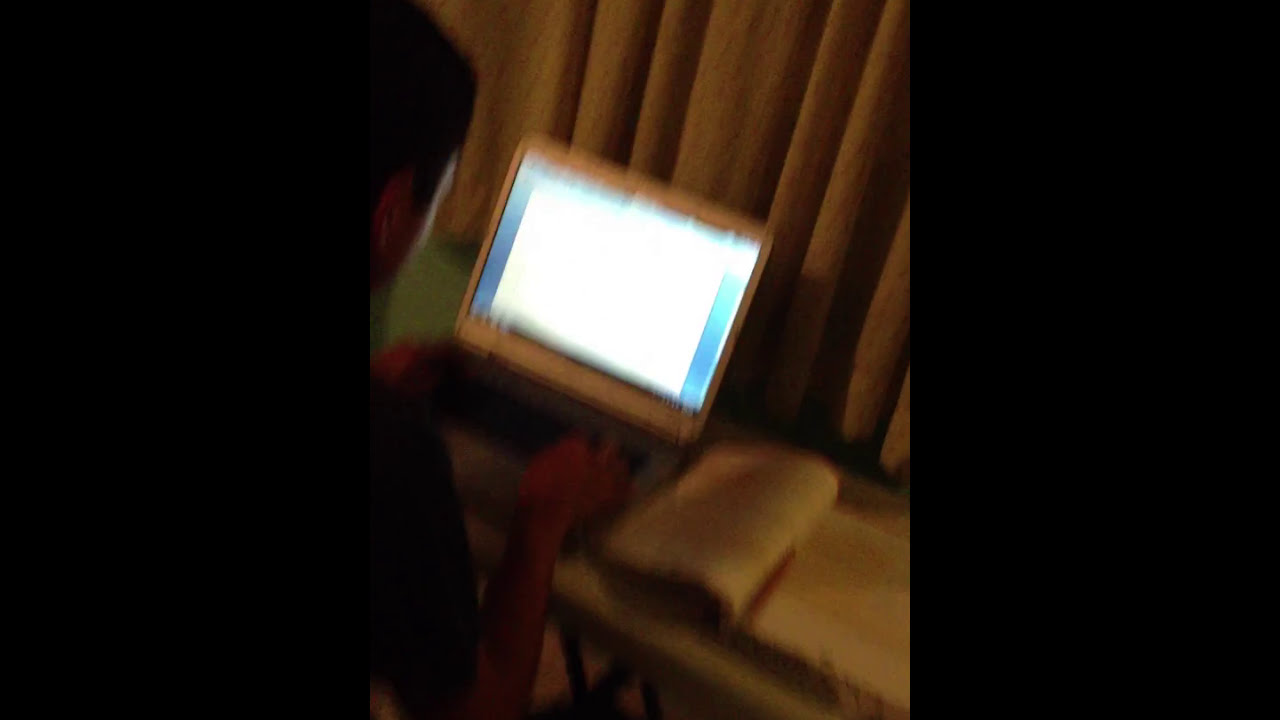The image is a vertically-oriented, blurry photo, possibly a still frame from a video or a low-light capture, depicting a boy sitting at a desk using a laptop. The screen of the light-colored laptop is on, showing a blue background with a prominent white box in the center. The boy's hands are positioned on the keyboard, and he is partially visible, wearing a dark-colored shirt. To the right of the laptop, an open book or notebook lies with a red pencil resting in the fold of the pages. Behind the laptop, there are closed tan curtains. The image has thick, solid black bars on both the left and right sides, serving as borders.